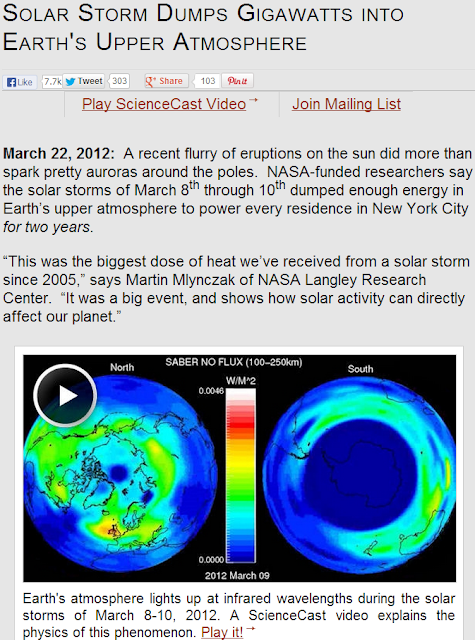This composite image vividly captures the significant impact of a solar storm that deposited gigawatts of energy into Earth's upper atmosphere in March 2012. Centered within the image is Earth, where discernible continents are mapped against a backdrop of vibrant colors—green, aqua, yellow, and blue—indicating varying intensities and effects of the storm. 

On the left side, the Northern Hemisphere is depicted with a prominent scale marked "Sabre No Flux, 1 to 250 kilometers," providing context for the spatial dimensions of the event. The date, March 9th, 2012, is prominently displayed, situating the viewer within the temporal framework of the occurrence. 

To the right, the Southern Hemisphere is shown, predominantly in shades of blue, with regions that possibly represent Antarctica or Australia accented by patches of aqua and bright green. 

A brief annotation beneath the image contextualizes the phenomenon: "Earth's atmosphere lights up at infrared wavelengths during the solar storms of March 8th to 10th, 2012." Additional text references a science cast video that elucidates the underlying physics of this breathtaking display, encouraging viewers to deepen their understanding of this natural event.